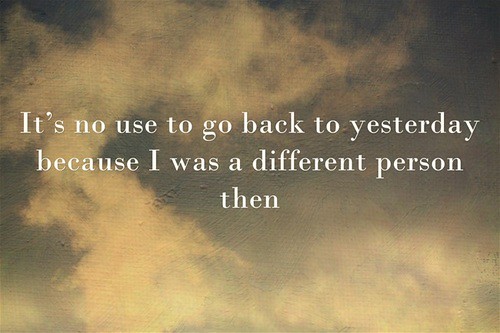The image features a sky with a brownish, yellowish tint that deepens to a darker hue in the top right corner. The background appears almost painted, with fluffy white clouds spreading from the bottom right corner up to the lower left and across the top. The central area and upper right corner are devoid of clouds, contributing to the image's dark and atmospheric feel. Overlaid on this sky backdrop is an inspirational quote in white text: "It's no use to go back to yesterday because I was a different person then." The text is arranged with the line "It's no use to go back to yesterday" at the top, followed by "because I was a different person", and ending with "then" at the bottom. The overall impression is of a poignant piece designed to evoke an emotional response, enhanced by the clouded, almost vintage-paper appearance of the sky.